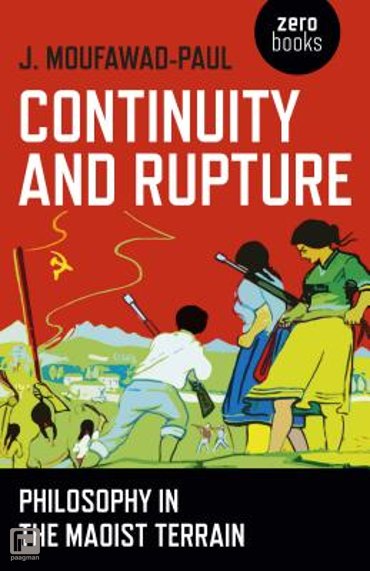The image is a book cover for "Continuity and Rupture" by J. Mufawad-Paul. The title is prominently displayed with the author's name at the top. The design features a Chinese flag being waved, and there are several people, including women and men, holding guns, suggesting a revolutionary or wartime theme. The background is primarily red to match the Chinese flag, transitioning into other colors such as green, yellow, blue, and brown towards the bottom. The text "Philosophy in Maoist Terrain" is displayed on a black background with white letters at the bottom of the cover. There is a circular logo at the top that says "Zero Books," indicating the publishing company. The overall composition suggests a detailed and vivid portrayal of Maoist revolutionary themes.